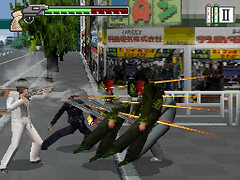A screenshot from a video game reminiscent of the PlayStation 2 era is depicted. The graphics evoke a nostalgic, yet not entirely retro, aesthetic typical of that period. In the upper right corner, a Roman numeral II is displayed in black lettering on a white scroll, accompanied by two similar scroll images. Central to the snapshot is the detailed image of a gun, showing the handle, trigger, and main body, as well as a health bar that extends from the barrel and alternates between green and red. In the foreground, three to four characters in black and gray attire appear to be collapsing, affected by being shot. The action reveals streaks of orange emanating from a shotgun, which is wielded by a figure dressed entirely in a white suit.